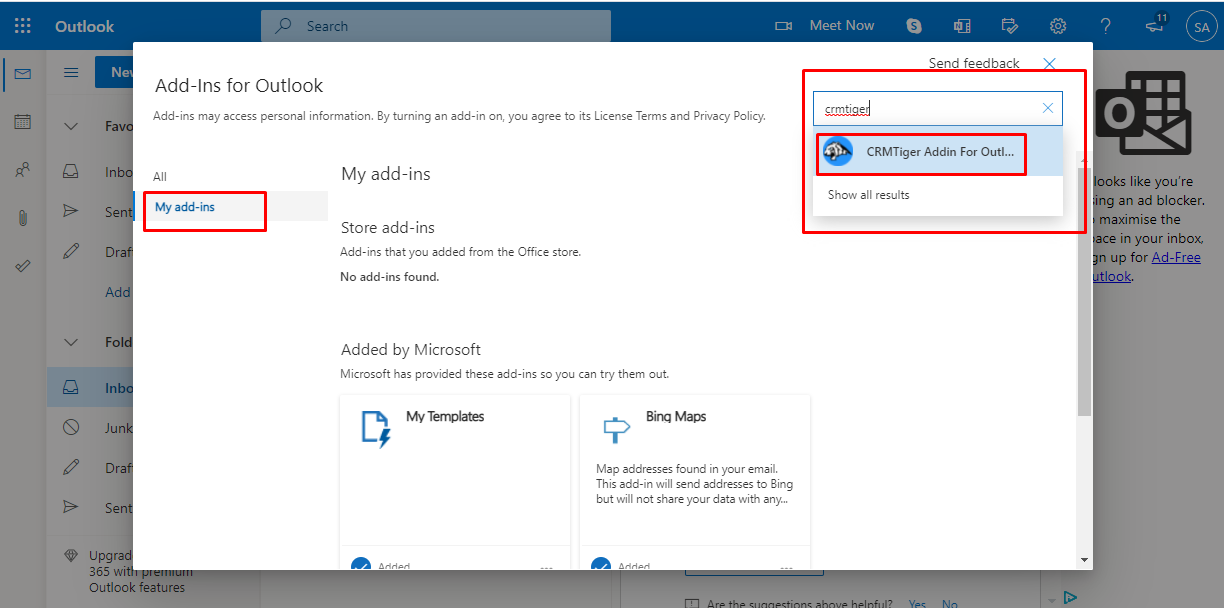A screenshot captured from a computer screen displays the Outlook web page in the background. In the foreground, a pop-up window titled "Add-ins for Outlook" has appeared, likely triggered by an action from the user. The pop-up window conveys important information about add-ins, stating, "Add-ins may access personal information. By turning an add-in on, you agree to its license terms and privacy policy."

As you scroll down this pop-up window, you encounter several sections. The first section, "My add-ins," indicates that no add-ins have been found. The next section, "Store add-ins," lists add-ins that you can add from the Office Store. Below that, a section titled "Added by Microsoft" informs users that Microsoft provides some add-ins for trial purposes. Examples of such add-ins include "My Templates" and "Bing Maps," both marked with a checkmark that signifies they have been added.

On the left side of the pop-up, the word "All" is visible, with a prominently drawn red or orange rectangle around the "My add-ins" section. In the upper right corner of the window, another red rectangle highlights a text box labeled "CRM Tiger add-in for Outlook..." indicating where users can type or search for specific add-ins.